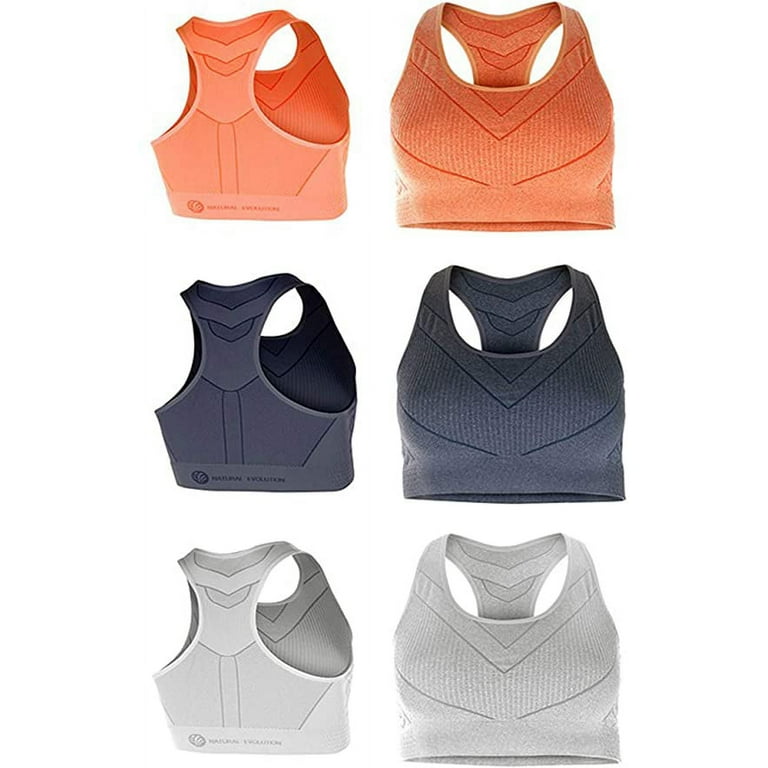This image displays a professionally taken, white-background collection of sports bras presented for an online shopping website. The layout consists of three rows, each showcasing the same sports bra model from both the front and back angles. The bras are presented in three different colors: the top row features a light peach or orange bra with subtle red highlights, the middle row displays a dark navy blue bra, and the bottom row offers a light grayish-white option. Each bra is depicted with detailed clarity, highlighting their lightweight, comfortable design suitable for activities such as running, yoga, or weight training. The images emphasize the feminine and practical nature of the garments, though the brand logo remains too small to identify. There is no definable border around the image, creating a floating effect typical of e-commerce product presentations.